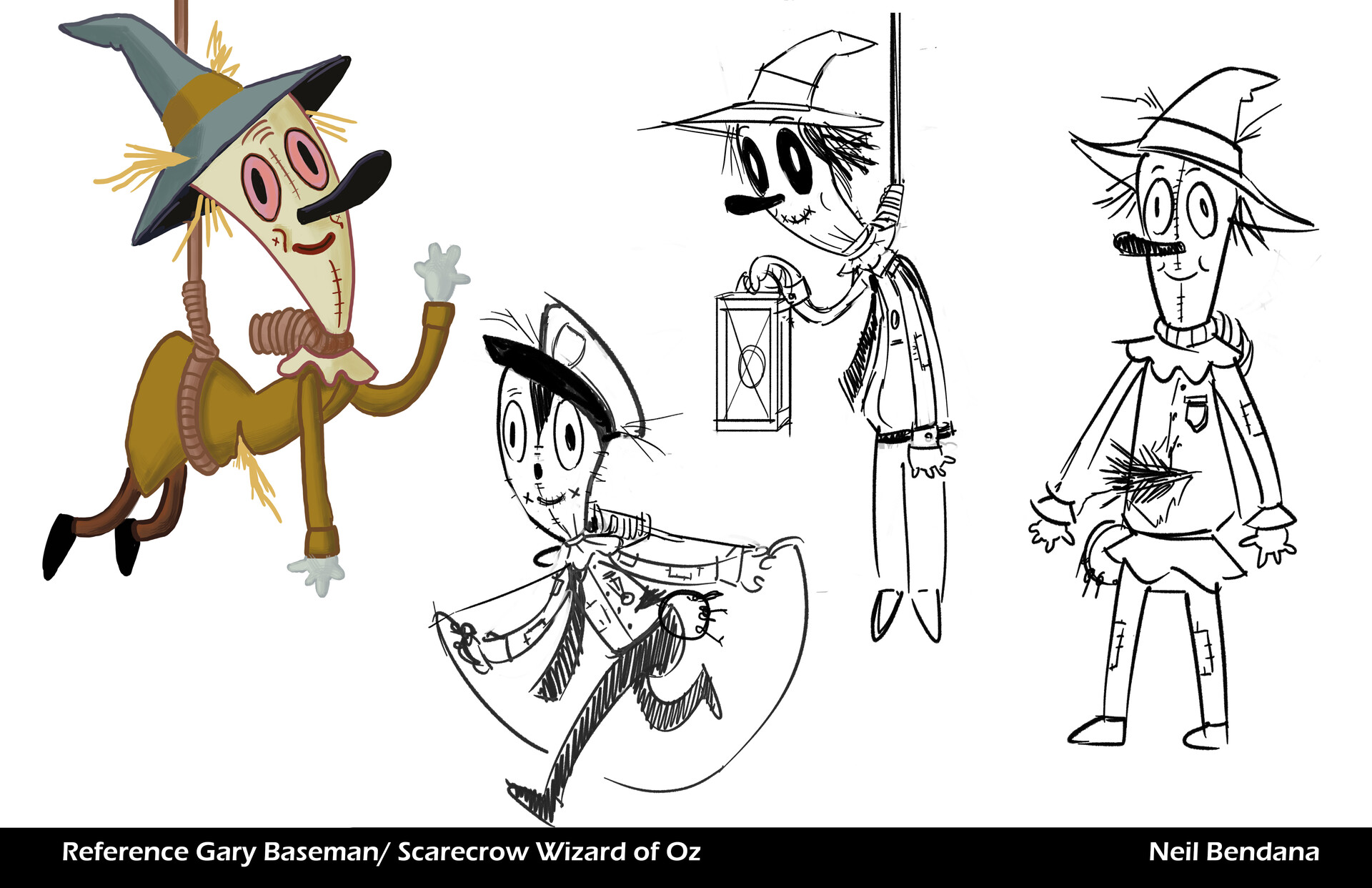This detailed illustration, referencing Gary Baseman and Neil Bendana's interpretation of the Scarecrow from "The Wizard of Oz," features four distinct character depictions against a white background. 

1. On the far left, a colorized Scarecrow stands out, wearing a black witch's hat with hay protruding from underneath. Dressed in a brown ensemble with a darker, brick-red belt, it has notably pink eyes with black centers and a prominent long black nose.

2. Next, a black-and-white sketch depicts a Scarecrow dressed as a policeman, complete with a cape. Underneath the cape, a large ring of keys adorns its belt. It has dark circles around the eyes and a pronounced black nose, exuding an authoritative presence.

3. To the right, another Scarecrow appears, hanging by a noose around its neck. Clad in a long-sleeve top and pants, it clutches a lantern in its right hand. The detailed facial features, including a grey witch's hat and dark rings around its eyes, emphasize its grim appearance.

4. The final Scarecrow stands quietly, donning a black witch's hat with hay sticking out. It features a large black Pinocchio-like nose and wears a long-sleeve jacket with a badge on the upper left side, evocative of an official or authoritative figure.

At the bottom of the illustration, a black rectangle with white writing states: "Reference Gary Baseman / Scarecrow, Wizard of Oz. Neil Bendana." This text complements the varied and imaginative portrayals of the classic Scarecrow character, emphasizing their unique details and diverse interpretations.